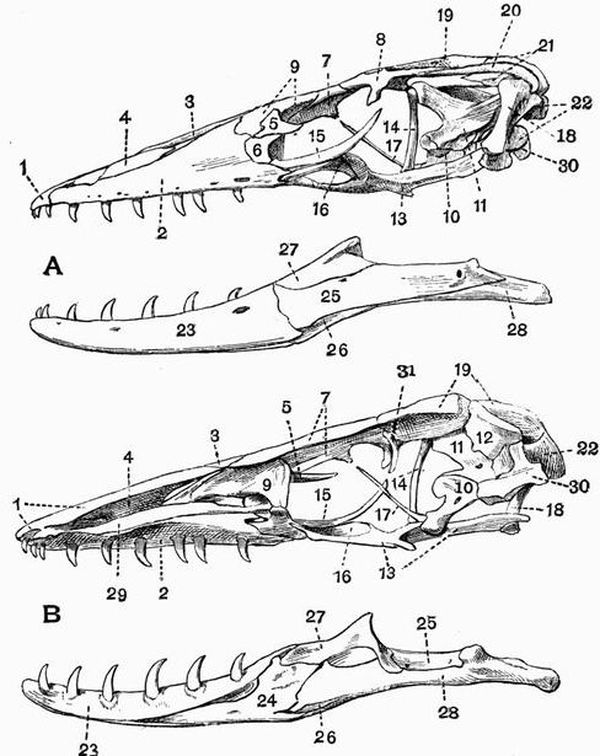The image is a vertical, rectangular diagram with a white background, featuring four detailed black and white sketches of jawbones, possibly from a reptilian creature like a dinosaur, crocodile, or shark. The diagram is divided into two main sections, each illustrating the top and bottom parts of an animal's mouth, arranged vertically from top to bottom. Each jawbone is meticulously labeled with numbers, starting from 1 on the left tip and escalating to 30 on the exterior curve, detailing various anatomical parts. The upper section displays bones that are narrow on the left and widen to the right, characterized by teeth along the front, hinting at an upper jawbone. This section is labeled with numbers, methodically increasing from 1 to 22, and then jumping to 30. Beneath it, there are another set of bones labeled from 23 to 28. The bottom section mirrors the structure of the top, with slightly thicker bones and more prominent teeth, numbered from 23 upward. The illustrations do not feature any descriptive text, only numerical labels that annotate different bone sections. The entire layout suggests a detailed anatomical study likely used for medical or educational purposes, emphasizing the intricate structure and comparative anatomy of the jaws.